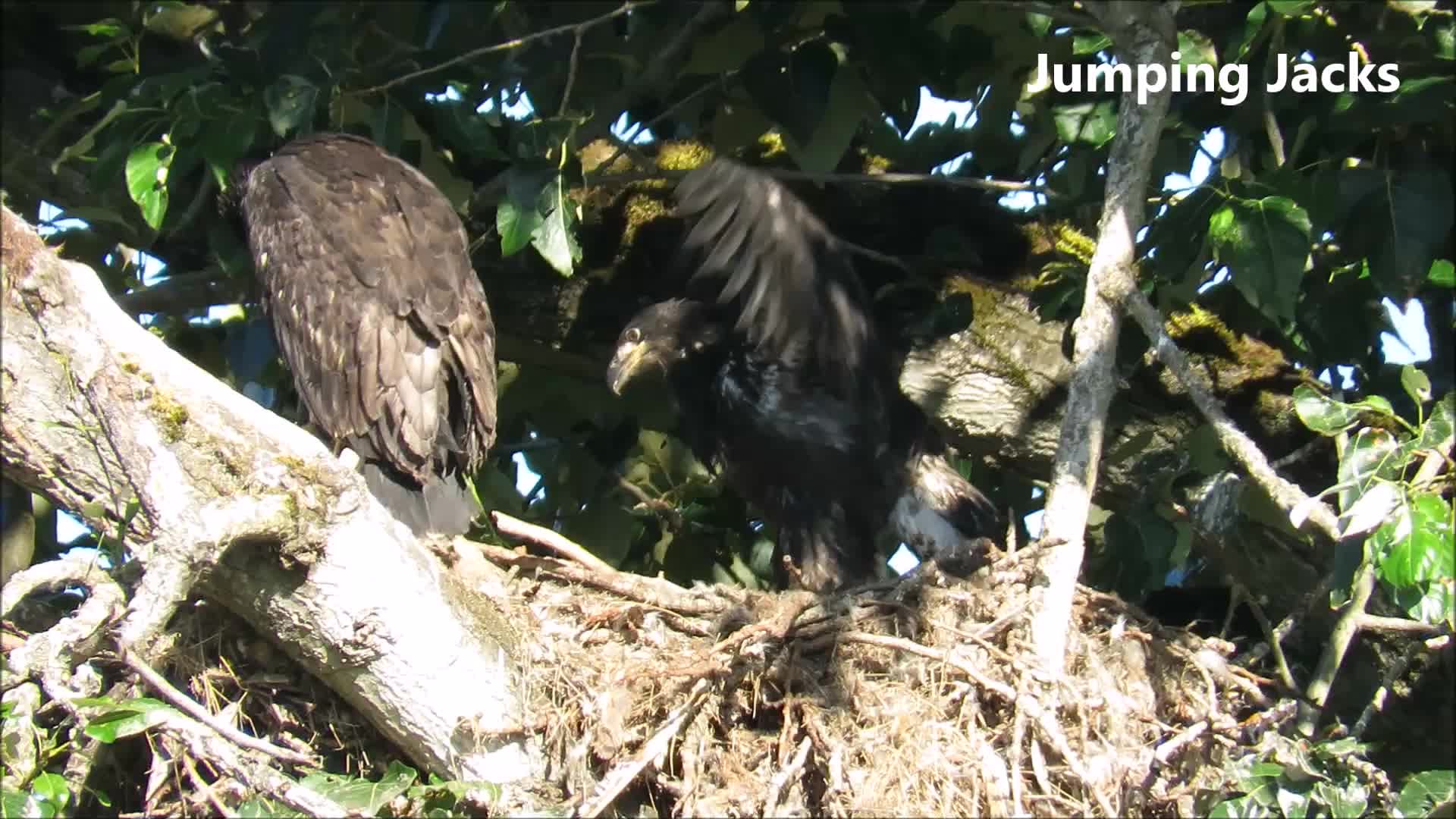The image is a detailed wildlife scene set in a vibrant, leafy thicket or tree. Prominently featured are two large birds perched on branches near a sizable bird's nest composed of twigs and straws, located at the bottom right. One of the birds, on the left, displays brown feathers, though its head is obscured by a large white branch extending upward and off the image. To the right of this bird, another bird with prominent black feathers can be seen more clearly, including its head and long beak. Behind these birds, another large branch runs diagonally from the bottom right to the upper left, intertwining with the dense green foliage and smaller branches. The backdrop reveals a bright blue sky peeking through the lush leaves, emphasizing the daylight setting. In the upper right corner of the image, white text reads "Jumping Jacks," adding a distinct caption to the scene.